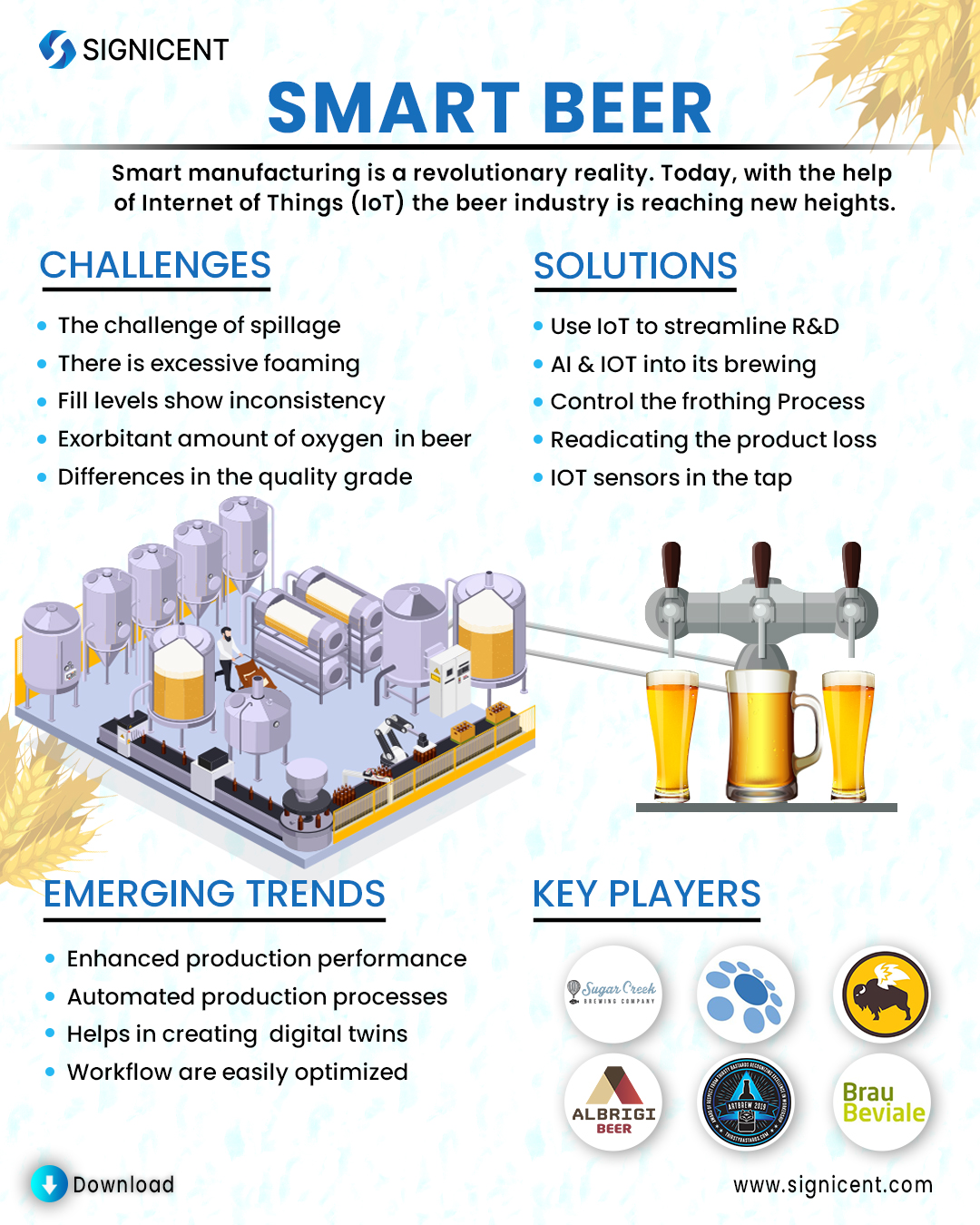This detailed vertical rectangular flyer titled "Smart Beer" on a white background with predominantly black text and all caps blue titles, explores the transformative impact of smart manufacturing on the beer industry. The title "Smart Beer" is prominently displayed in large blue letters, underlined in black, with the subtitle reading, "Smart Manufacturing is a Revolutionary Reality. Today with the help of Internet of Things, the beer industry is reaching new heights." At the top left, there's a blue emblem next to the word "Signescent" and on the top right, a graphic of gold-colored leaves on branches.

The flyer is divided into four main sections, each with a heading in all caps blue letters, underlined in black. The top left section, titled "CHALLENGES," outlines various industry issues such as excessive foaming, inconsistent fill levels, excessive oxygen in the beer, and quality grade disparities, listed with black text next to blue bullet points. To the right, under the heading "SOLUTIONS," it discusses how smart manufacturing addresses these challenges with detailed bullet points.

Central to the flyer are two key illustrations: on the left, a factory design, and on the right, a spout pouring beer into three glasses. At the lower part of the flyer, the left section titled "EMERGING TRENDS" elaborates on advancements like enhanced production performance, automated processes, digital twins, and optimized workflows. The bottom right section, "KEY PLAYERS," features six circles, each containing logos and names of the companies driving these innovative changes.